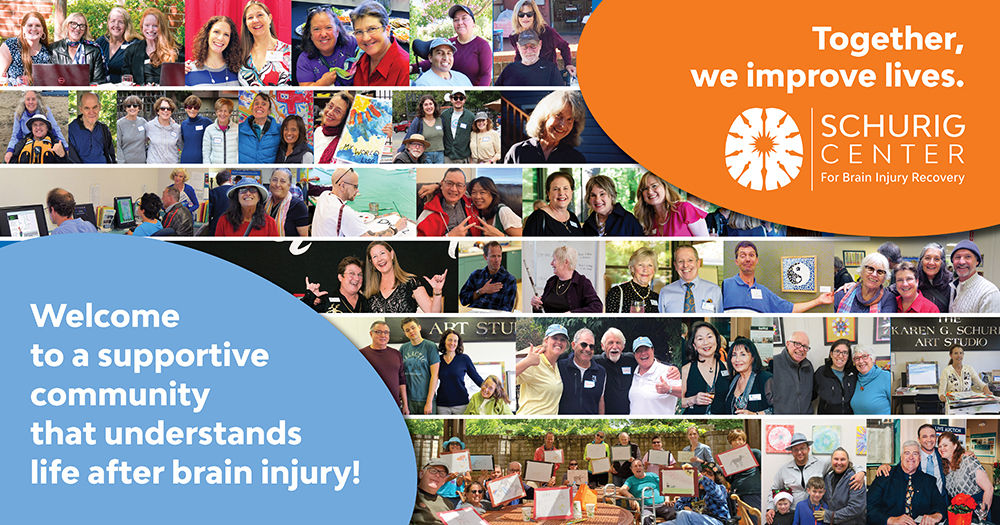This advertisement for the Schurig Center for Brain Injury Recovery prominently features a mosaic of images displaying six rows of patients, medical personnel, and groups of people engaging in various activities such as holding signs, giving thumbs up, and attending lectures. The collage, which showcases individuals and groups celebrating and smiling at the camera, conveys a sense of community and support. In the upper right-hand corner, a distinct orange oval contains the text: "Together, we improve lives," alongside the center’s name and a white illustration of a brain. The lower left-hand corner features a quarter blue oval with the message: "Welcome to a supportive community that understands life after brain injury." This vibrant and detailed composition collectively highlights the center's dedication to recovery and community.